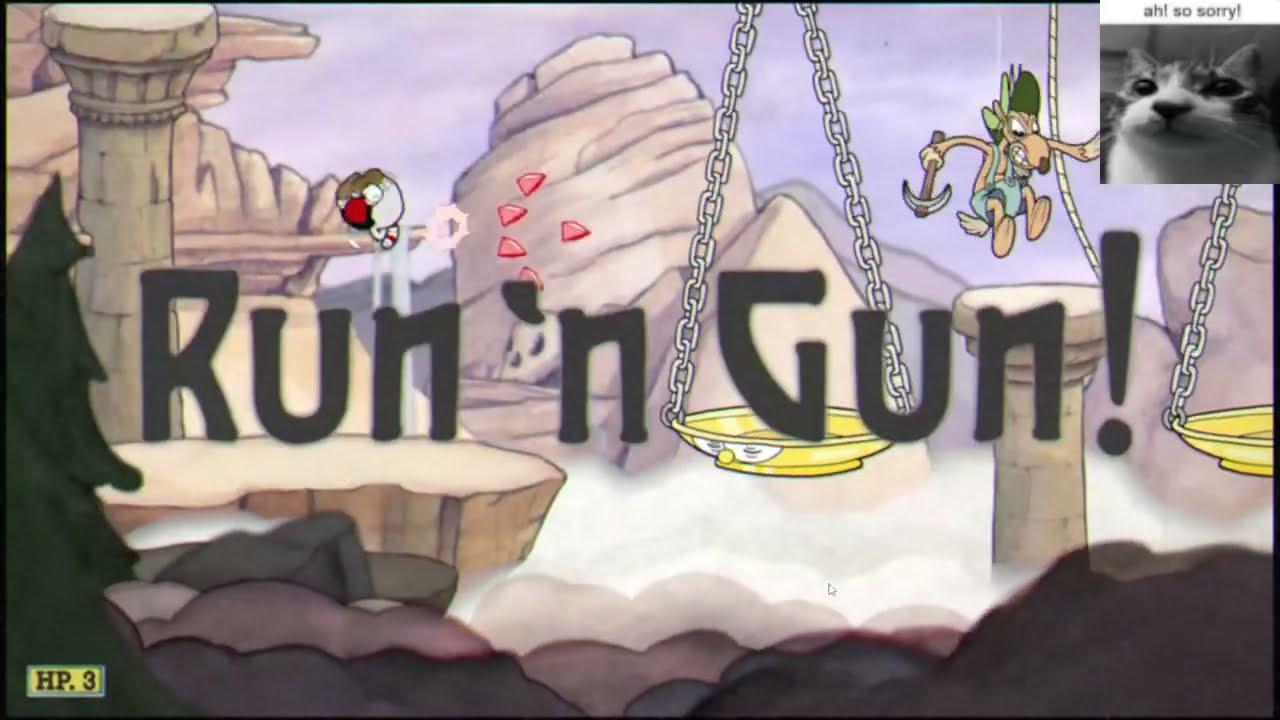This detailed rectangular screenshot from the video game "Cuphead" captures a vivid scene brimming with action and visual nostalgia. The horizon is painted a serene lavender, dotted with clouds, and encircled by various beige rock formations and distant mountains. In the foreground, on the bottom left corner, stands a tall green tree. A flat beige rock surface stretches across the bottom, dominated by dark gray, cloud-like objects. From this surface, a column, reminiscent of a Greek pillar, projects towards the top left corner.

Central to the image is the main character, Cuphead, dynamically jumping and spiraling up mid-air, clad in his iconic white hat, brown shoes, and sporting a red-and-white striped straw from his head. He energetically shoots small, sharp red projectiles. Perched amid the action is a coyote prospector character, equipped with a pickaxe, wearing overalls and a green hat. Hovering in the air, this coyote seems to be the target of Cuphead’s barrage. 

Enhancing the scene’s characteristic charm, two gold plates hang from chains on the right side, with one plate prominently reading "Run and Gun" in bold gray type. Adding a quirky touch, a black and white photo of a cat with the label "LR!" is nestled in the upper right corner. This screenshot is a perfect encapsulation of "Cuphead’s" distinctive blend of vintage animation style and fast-paced gameplay.